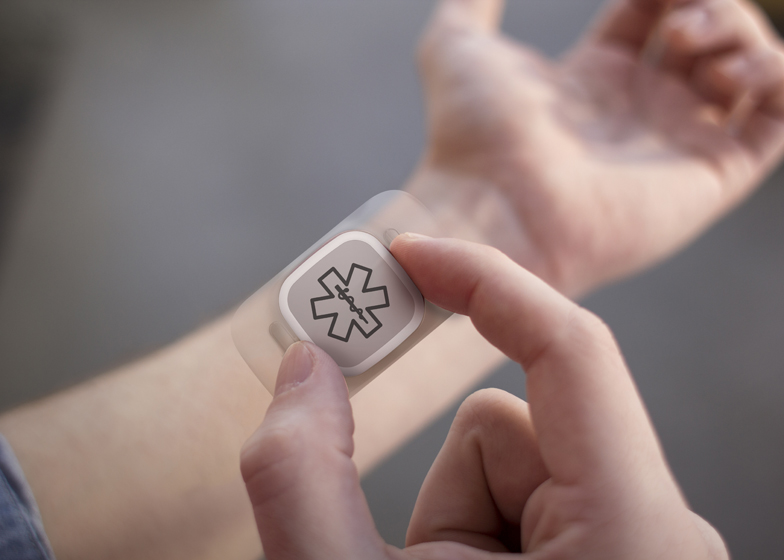The image features a photorealistic representation of a person's hands against a gray background. In the foreground, a right hand is prominently displayed, holding a clear and white rectangular device with a caduceus emblem and a six-pointed cross. The right hand's thumb and index finger are gripping the device, which appears to be a medical alert or adhesive medical device. The left hand, less focused and blurred, is shown from the forearm to the fingers, with its palm up and fingers slightly curled inward, as if preparing to receive the device. There is a hint of a denim shirt cuff on the left forearm. The detailed depiction creates the impression that the right hand is about to place the adhesive medical device onto the wrist of the outstretched left hand.